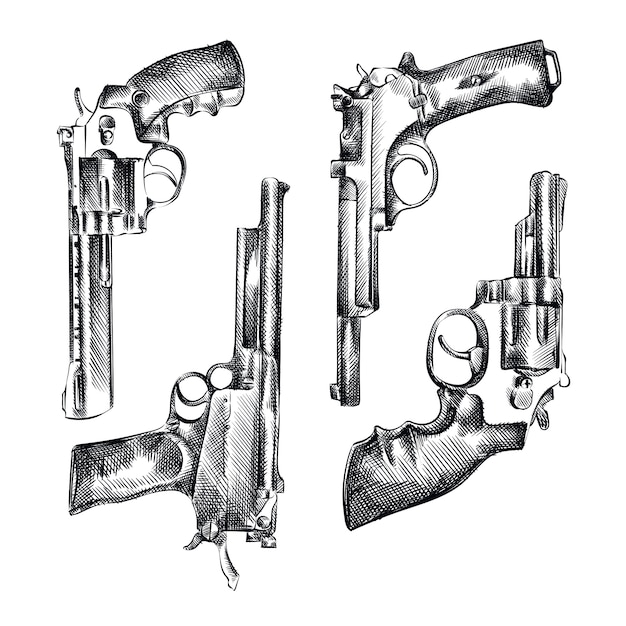This detailed pencil drawing features four different handguns meticulously arranged against a plain white background. The guns alternate in orientation, with the first pointing downward, followed by one pointing upward, then another downward, and finishing with one pointing upward. The first gun on the left is a revolver, recognizable by its distinctly curved pistol grip and downward-pointing barrel, likely a larger model like a .357 Magnum. The second gun from the left appears to be a Luger pistol, characterized by its upward-pointing barrel, a grip that likely houses the magazine, and a smooth profile. The third gun is another depiction of a Luger but with a slightly longer barrel and a distinctive screw on the grip, pointing downward. The final gun on the right is a smaller revolver with a snub-nose barrel, possibly a .38 special, also featuring a curved grip for ergonomic finger placement. Each firearm is rendered with careful attention to detail, showcasing the unique features and mechanical intricacies of each type, all set upon an unadorned, white backdrop that emphasizes their forms.